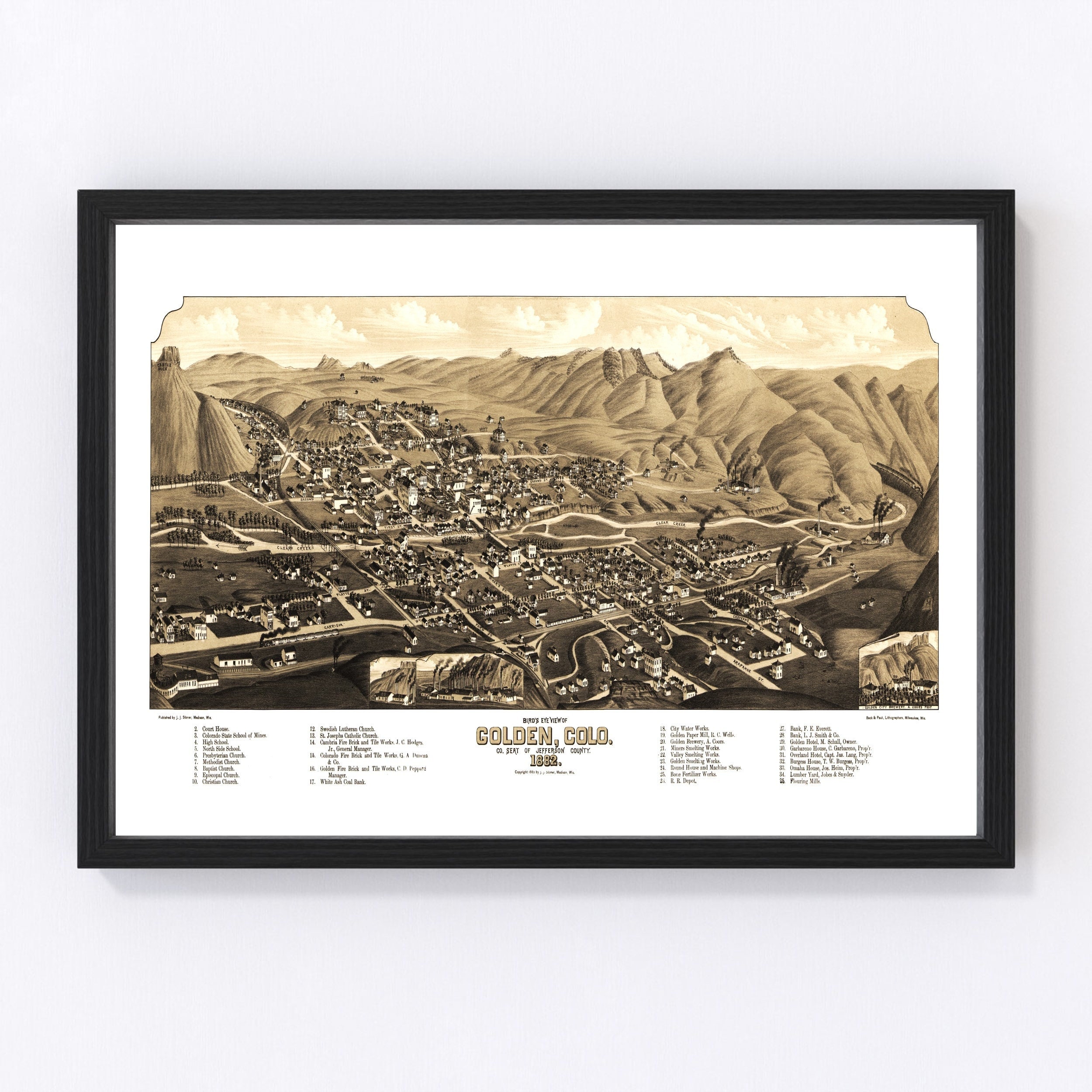This image features a historical, sepia-toned print titled "Golden, Colorado, Seat of Jefferson County, 1882," meticulously framed in a thin, dark wood frame with white matting. The picture illustrates a detailed cityscape of Golden, Colorado, set against a backdrop of mountains and a partly clouded sky. The image captures a three-dimensional representation of the town's street network, houses, and key buildings, each identified by small numbers corresponding to landmarks detailed at the bottom. The central village is depicted with white houses and brown and golden tones accentuating the landscape, particularly in the mountains and sky. The print is surrounded by small, seemingly illegible text, adding to the historical and intricate nature of the artwork.